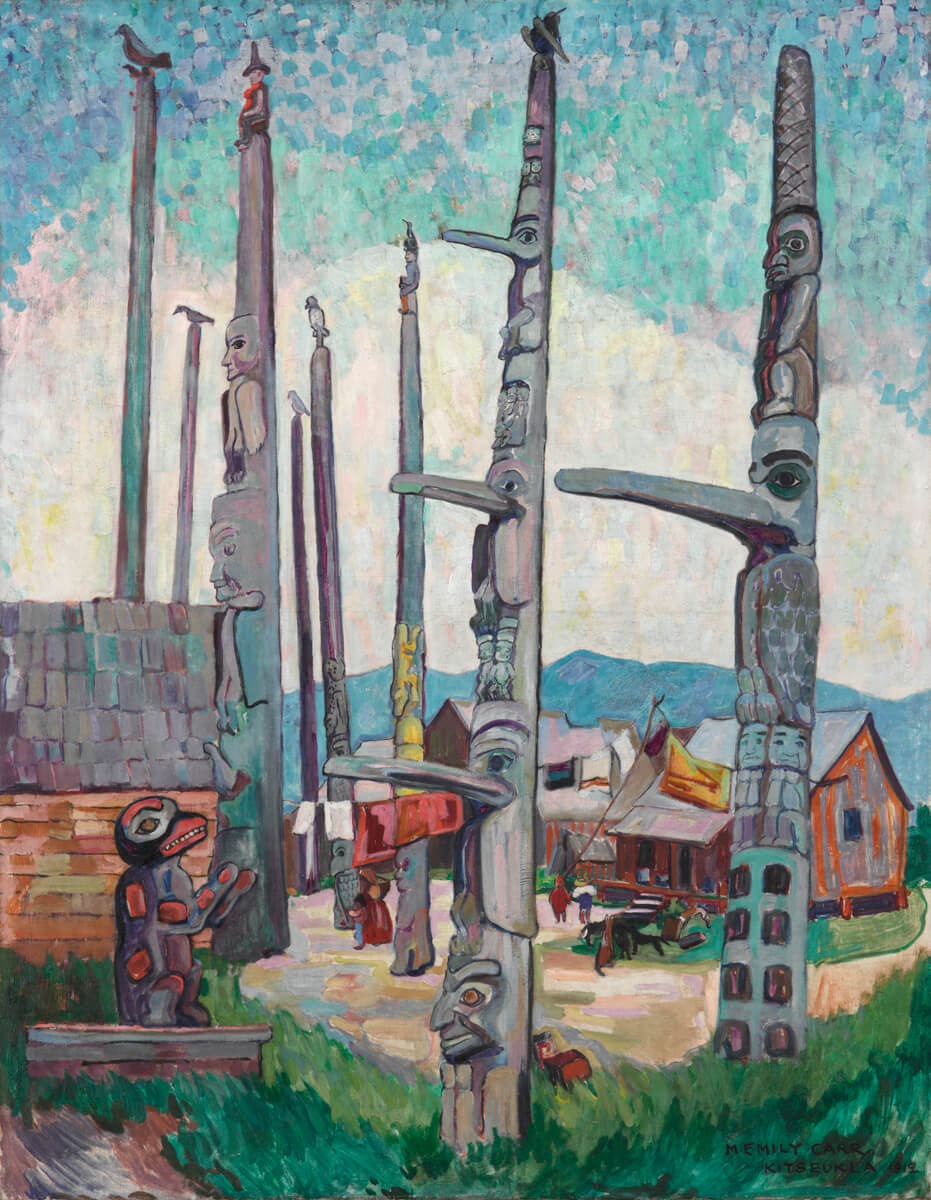The painting, titled "Totem Pole's Kitsukula" by Emily Carr, is a detailed watercolor scene featuring numerous tall totem poles adorned with intricate carvings. The totem poles, some painted in vibrant shades of yellow, red, and green, while others retain their natural wooden appearance, predominantly depict bird-like figures with prominent beaks. Set against a backdrop featuring a distant mountain view, the scene includes green grass covering the ground, a winding dirt or gravel path, and several small brown shacks on either side of the path.

In the foreground, on the bottom left, there's a curious figure resembling an animal, standing upright in a praying pose, gazing towards one of the totems. Adjacent is a white ledge over a red brick surface, partially obscured by grass, where another figure appears to be holding something and wearing a mask with large white eye areas and an orange top resembling a short beak-like mouth.

Notably, two crows perch on separate totems, and a person with a red scarf and a witch hat is intriguingly situated on another. The totem poles themselves are highly detailed compared to the rest of the softer, less-defined elements of the image.